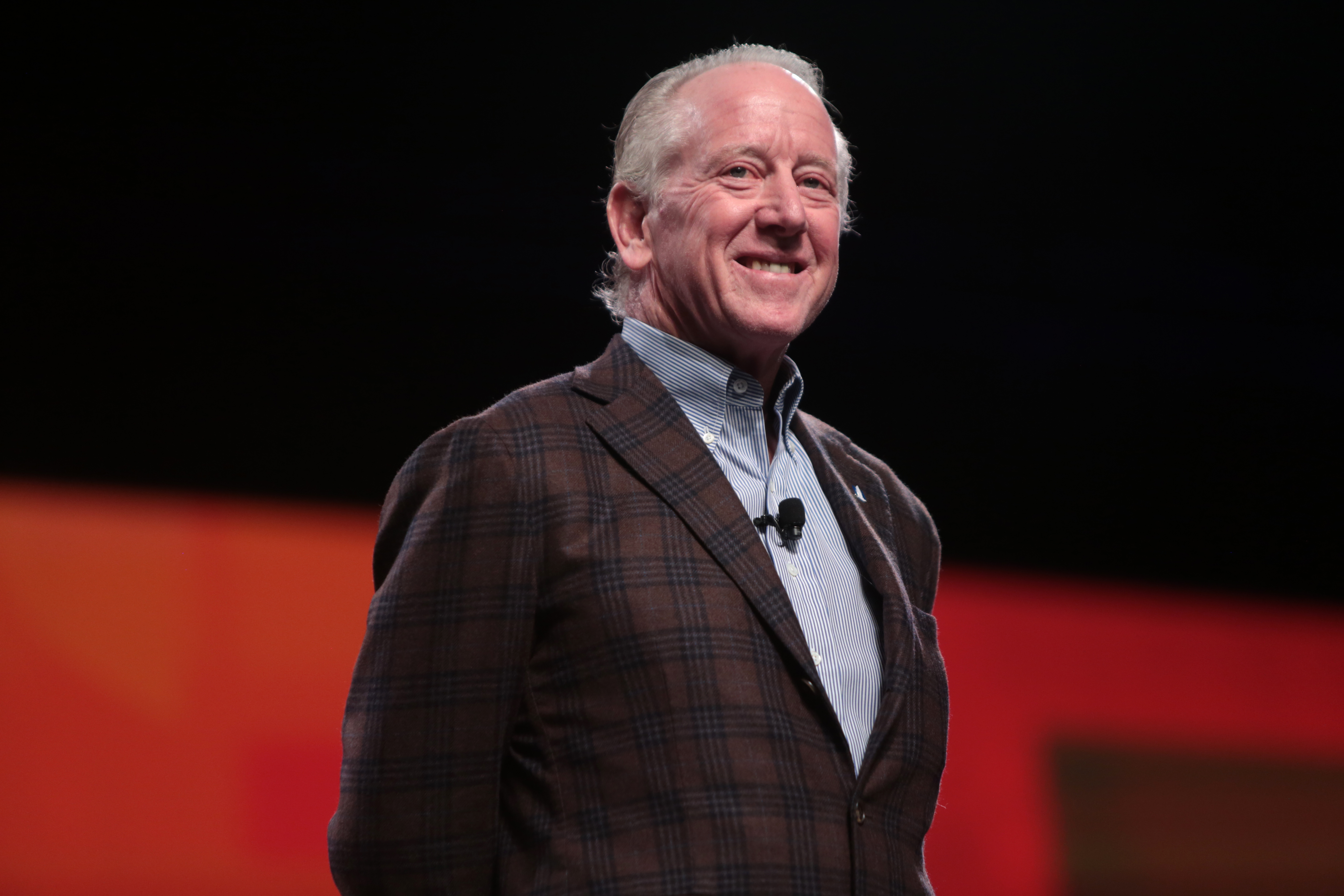This photograph captures an older white man, estimated to be between 70 and 80 years old, standing on a stage, presumably ready to give a speech. His well-lit figure stands out against a background that is blurred, with the upper part in black and the lower part in red, indicating a stage setting. He has slicked-back gray hair and some facial wrinkles, especially on the back of his cheeks, suggesting his advanced age. The man, who might be a former baseball player, stands confidently with his chest puffed out and his hands positioned behind his back. He is dressed in a checkered sports coat featuring a brown and blue plaid pattern over a blue and white striped button-down shirt with a collar. A small black microphone is clipped to his shirt, prepared to capture his speech. Despite not speaking yet, he is smiling, revealing some teeth, which creates a warm and approachable demeanor. The photo, taken from an audience perspective, frames him as the central and sole figure, emphasizing his prominence on stage.